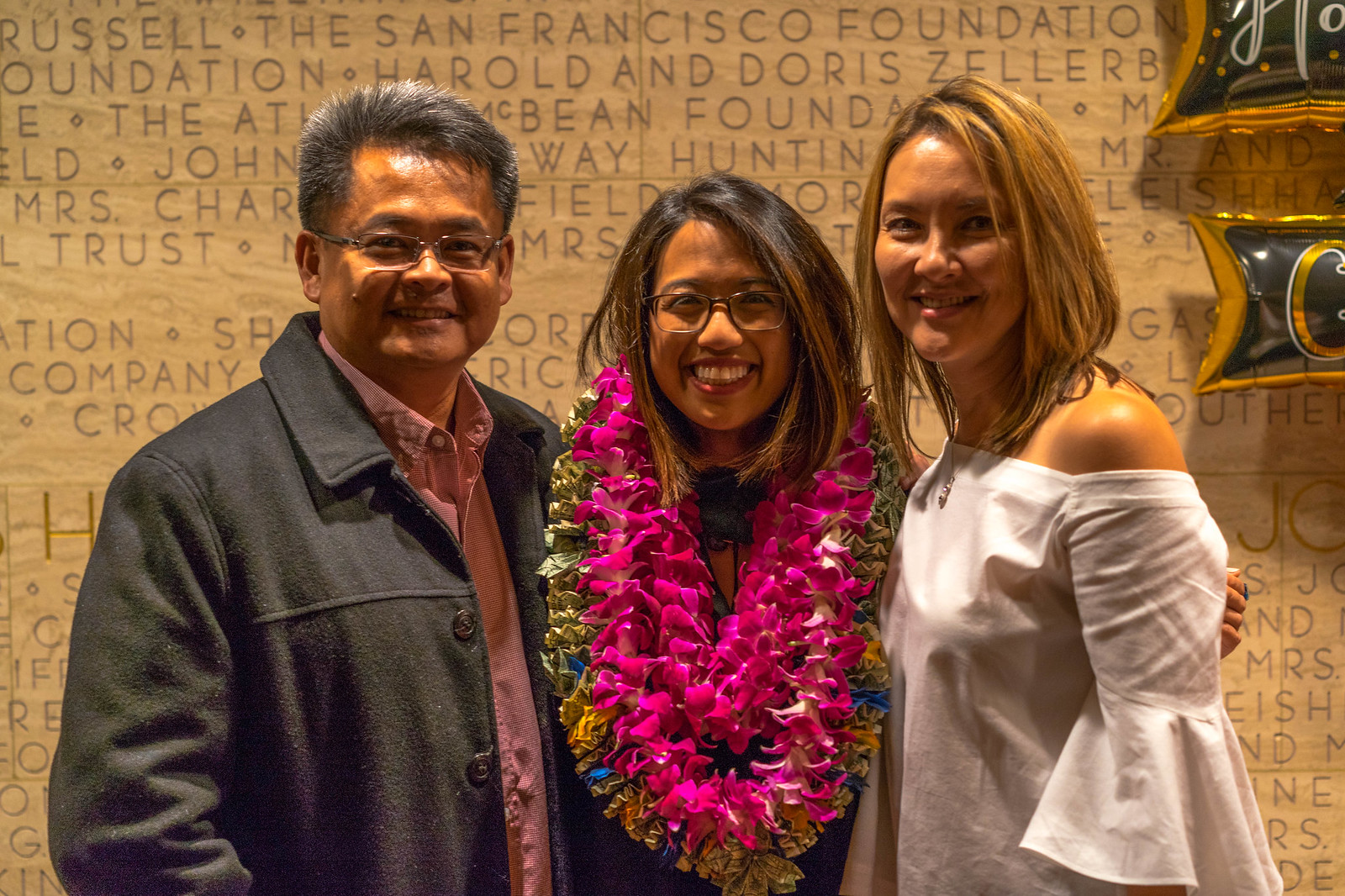In this image, a trio stands at the center, posing and smiling at the camera. The group consists of an older gentleman on the left, a woman of a similar age on the right, and a young lady in the middle. The man on the left, sporting slightly gray hair, glasses, a gray coat, and a light salmon-colored button-down shirt, has his arm around the young lady in the center. She is adorned with several pink and white flower leis. The woman on the right, dressed in a white top with fanned-out sleeves, also embraces the young lady. The backdrop features a stone wall with partially visible engravings, among which the text "The San Francisco Foundation" and names such as "Russell," "Harold and Doris," "Zeller," and "McBean Foundation" can be discerned. To the top right corner, a cluster of balloons suggests a celebratory occasion, likely taking place indoors. Color accents in the image include light brown, gray, maroon, brown, pink, purple, blue, gold, and yellow.